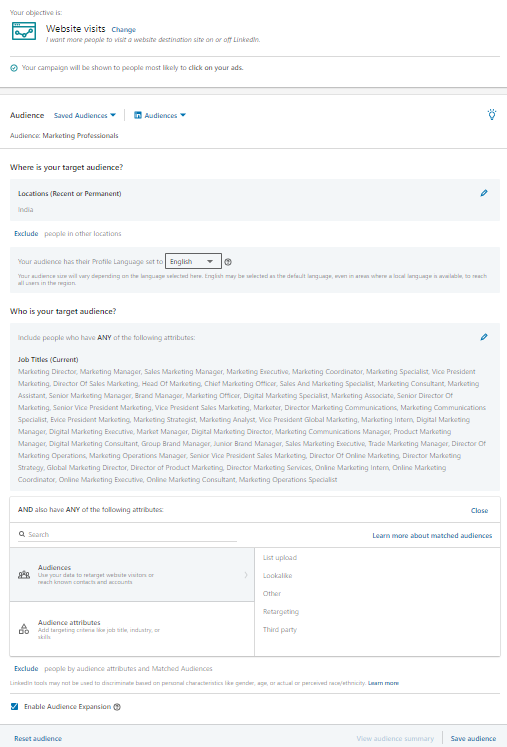The webpage features a layout where the content is displayed in small, difficult-to-read text, even when maximized. At the very top of the page, there is tiny gray text that reads, "Your objective is," followed by "Website visits" in black ink below it. To the right of this, the word "Change" appears in bright blue text. Underneath, in small gray italics, the text states, "I want more people to visit a website. Destination site on or off LinkedIn."

Directly below, there is a bright blue circle with a checkmark inside, accompanied by the message, "Your campaign will be shown to people most likely to click on your ads." A thin gray banner runs horizontally beneath this section. On a white background that follows, the word "Audience" is written in black text, with the phrase "Saved audiences" and a bright blue drop-down arrow located to the right. Below this, in gray text, it says "Audience marketing professionals," followed by another thin gray line running across the page. Further down, in black text, it asks, "Where is your target audience?" and the page continues with text that remains too small to be legible.